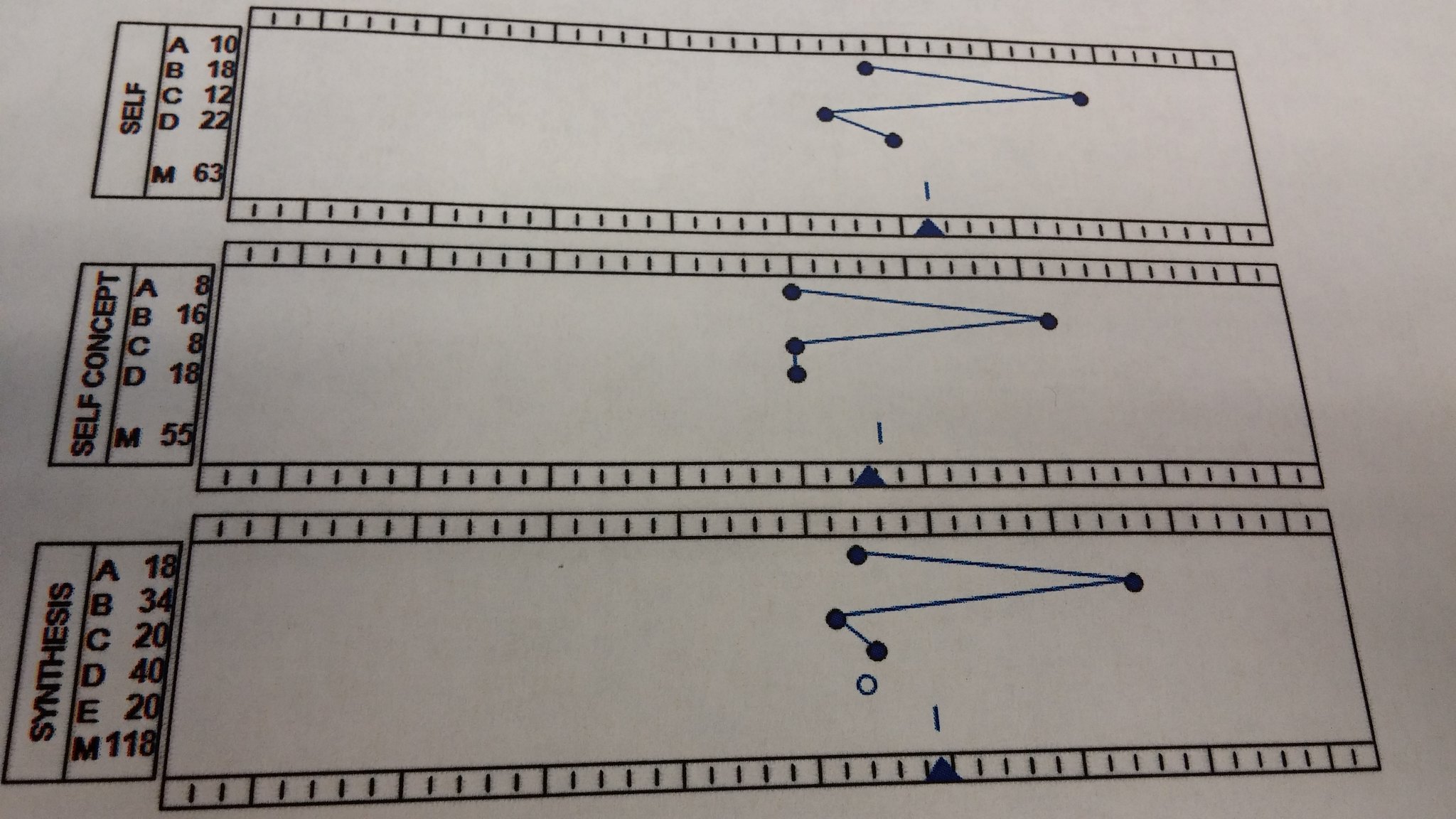This photograph features three distinct charts labeled "Self," "Self Concept," and "Synthesis," positioned from top to bottom respectively.

- **Top Chart (Self):** 
  - **Labels:** A, B, C, D, M
  - **Values:** 10, 18, 12, 22, 63
  - **Graph:** Displays a zigzag pattern resembling a "Z," prominently marked at specific points. Its purpose is unclear but it suggests some form of data monitoring.

- **Middle Chart (Self Concept):**
  - **Labels:** A, B, C, D, M
  - **Values:** 8, 16, 8, 18, 55
  - **Graph:** Exhibits a sideways "V" shape, comparable to a "greater than" (>) sign.

- **Bottom Chart (Synthesis):**
  - **Labels:** A, B, C, D, E, M
  - **Values:** 18, 34, 20, 40, 20, 118
  - **Graph:** Combines elements of a "greater than" (>) sign and a "Z," with a notable zero positioned near the zigzagging graph.

These charts collectively appear to track or analyze data points related to an unknown parameter, potentially aligning with aspects of well-being, mental health assessments, or lie detector tests.